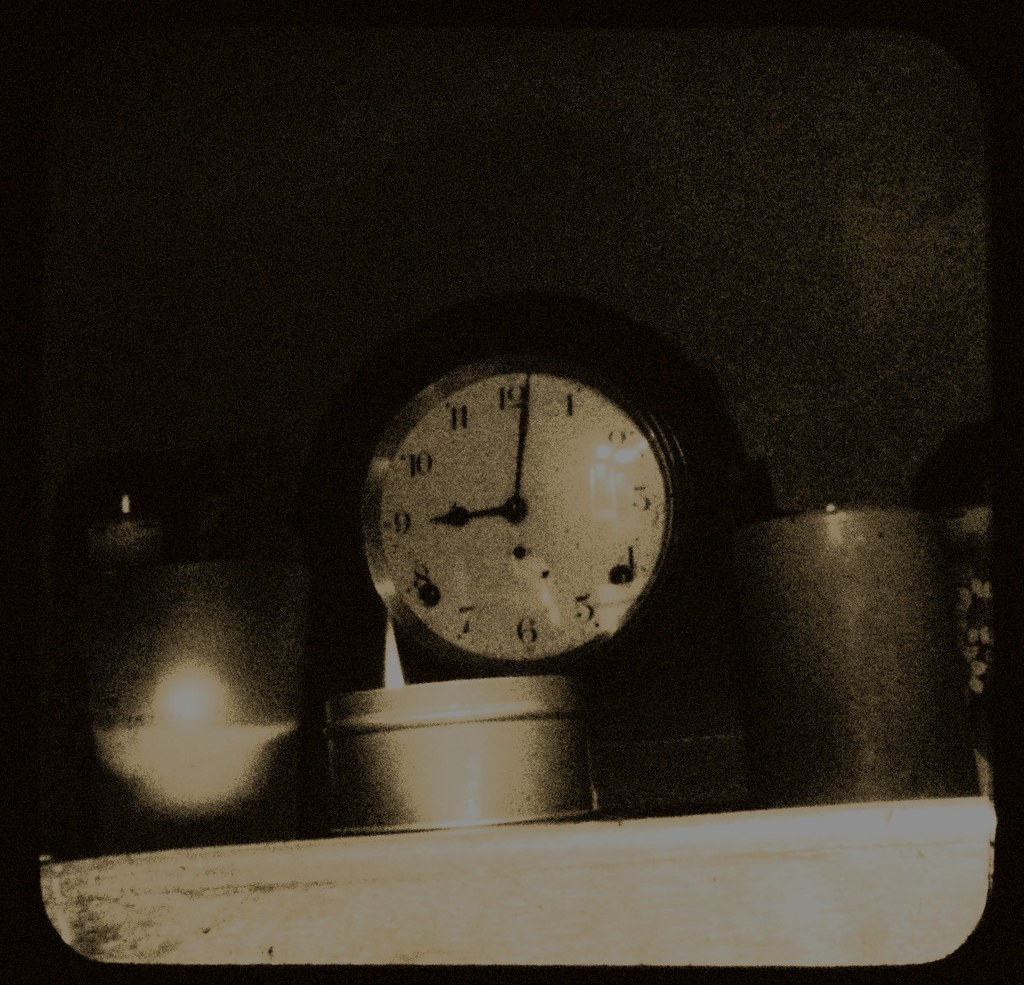In this grainy black and white photograph, a modest shelf serves as the base for an intriguing arrangement of objects. Atop the shelf sits a collection of three distinct candles. On the far left, a softly glowing candle emits a gentle light, suggesting it may be encased in a glass holder. The middle candle resembles a small tea light encased in a tin shell, with its flame flickering towards the left. To the right, a large cylindrical wax candle stands tall and sturdy. Behind these candles, a classic wooden half-moon clock, displaying the time as 9:01, adds an element of timeless charm to the scene. The indistinct wall in the background, shrouded in the graininess of the image, adds a sense of mystery and nostalgia, enhancing the vintage atmosphere of the composition.